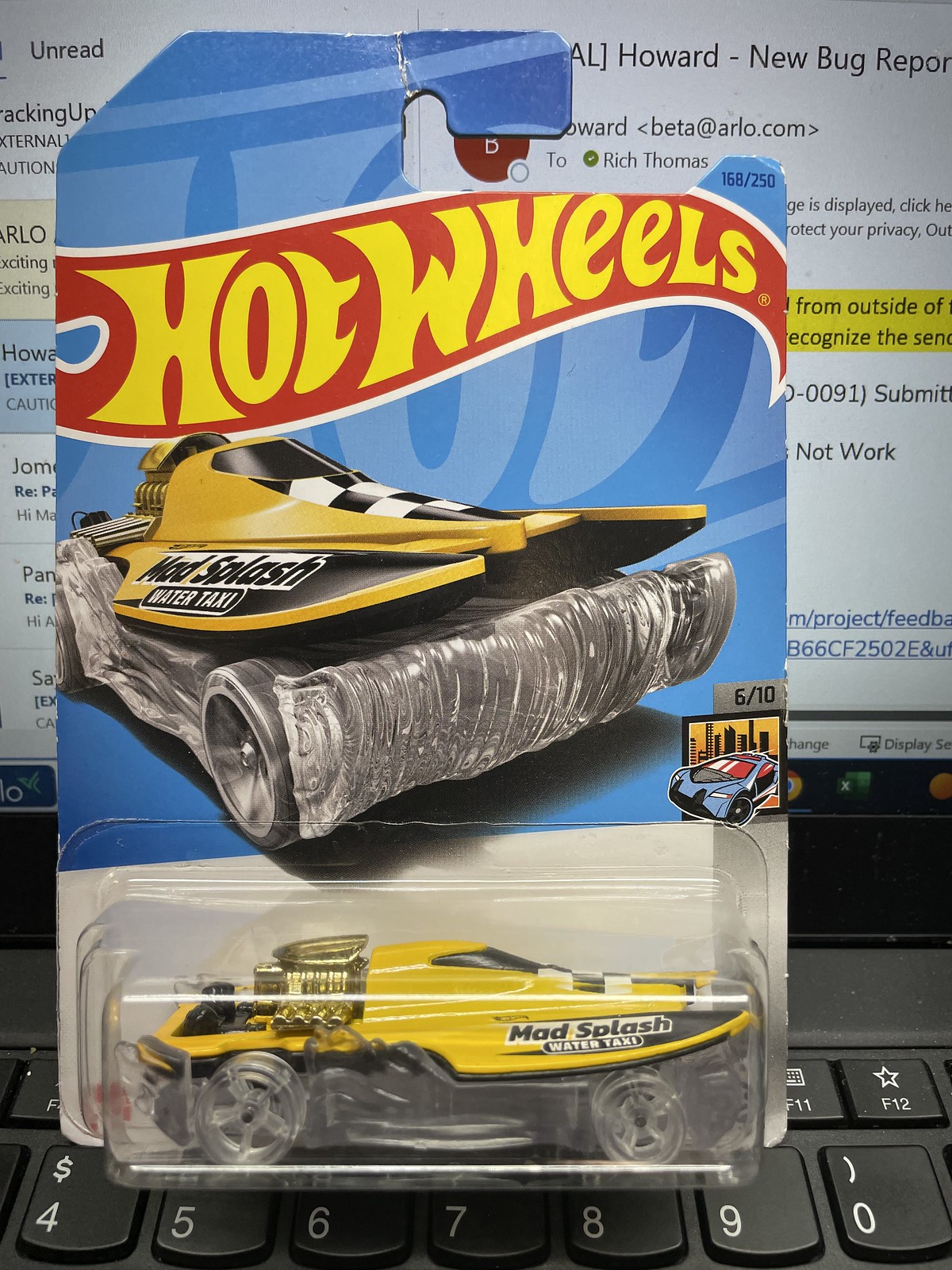The image captures a photograph of a Hot Wheels toy car, specifically the "Mad Splash Water Taxi," still enclosed in its original packaging. The vehicle is predominantly yellow with a black and white checkerboard pattern on top and a silver-hued underside. The packaging prominently displays the iconic Hot Wheels logo in yellow with a flame motif on a red background, set against a blue cardboard backing. Positioned just above the toy, the packaging indicates that this is number 6 in a series of 10, with an additional label marking it as 168 out of 250.

The "Mad Splash Water Taxi" text is clearly visible on the side of the car. The toy itself features transparent plastic surrounding it, highlighting the vehicle's boat-like shape with a black and white engine at the back, detailed black markings at the front, and a checkered pattern in front of the windshield. The entire package appears propped up against the number keys (4-9) of a black laptop keyboard, with the screen in the background open to an email application titled the "Howard Neubauer Report." The overall scene combines bright colors including red, blue, yellow, black, white, and silver, creating a vibrant visual.